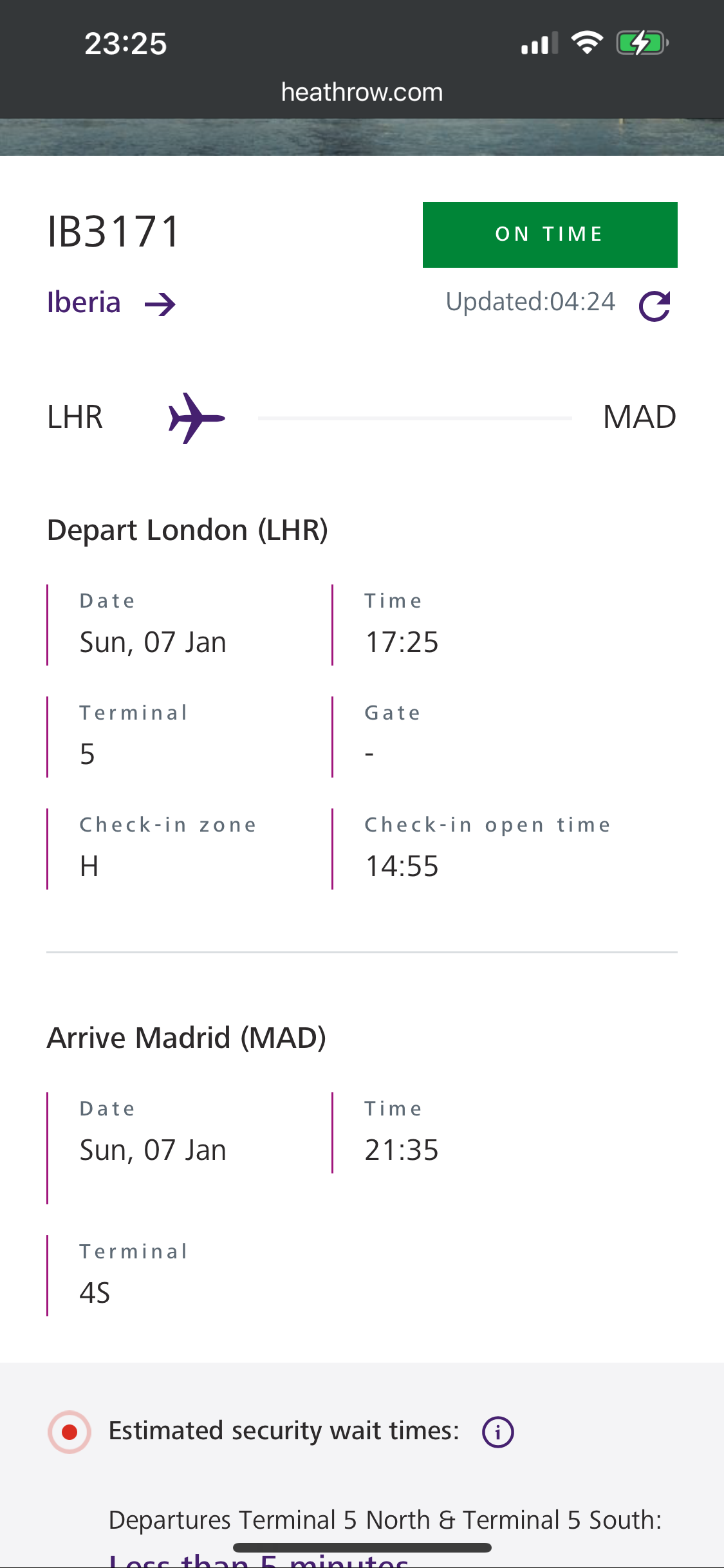Screenshot of the Heathrow.com website displayed on an iPhone with three bars of cell service, three bars of Wi-Fi, and a fully charged battery that is currently charging. The local time is 23:25. The screen shows flight details for IB3171 on Iberia Airlines, indicating the flight is on time, denoted by a green rectangle, with the last update at 04:24.

The flight departs from London Heathrow Airport on Sunday, January 7th at 17:25 from Terminal 5, with the check-in zone listed as H. Check-in opens at 14:55. The flight arrives in Madrid on Sunday, January 7th at 21:35, landing at Terminal 4S.

There is a section for estimated security wait times, which appears to be blank, accompanied by an information icon for more details. Below this, departure information for Terminal 5 North and Terminal 5 South is provided, indicating a wait time of less than five minutes.